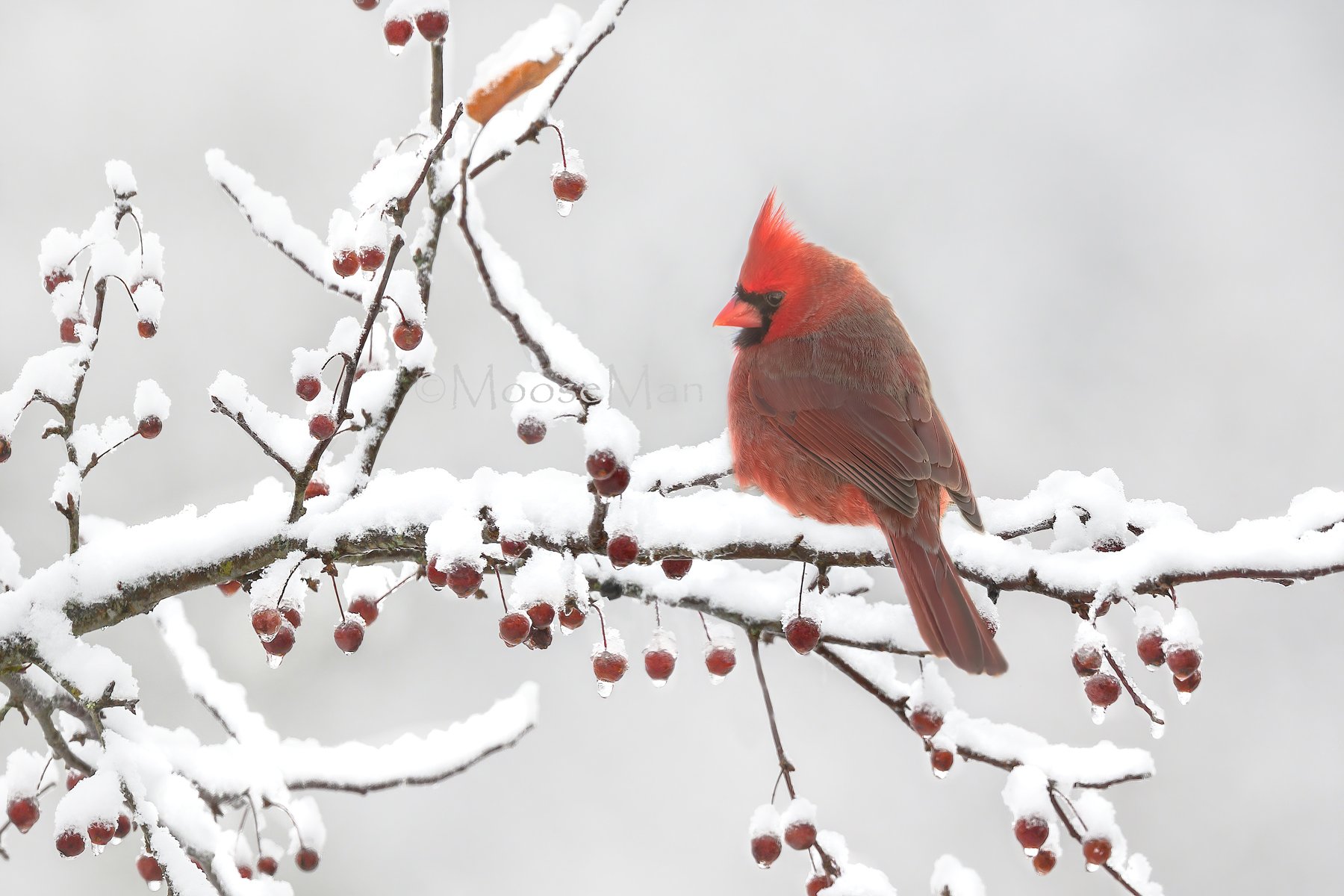A striking cardinal perches gracefully on a snow-laden tree branch, presenting a vivid contrast against the wintry backdrop. The cardinal boasts a vibrant red crest atop its head, a defining feature that complements its short, red-tipped beak. Its face is adorned with a conspicuous black mask which accentuates the brilliance of the red plumage. The bird's feathers transition to a more subdued brownish hue down its back extending to its tail. Its underparts are a blend of red and light brown tones.

The scene suggests a cherry tree, as evidenced by the presence of cherries hanging from the branch, each fruit encased in a delicate layer of ice, adding a crystalline shimmer. The branches themselves are heavily coated with fresh snow, creating an enchanting wintry tableau. The cardinal, seemingly unfazed by the cold, gazes serenely to the left, adding a touch of warmth and life to the frosty setting.